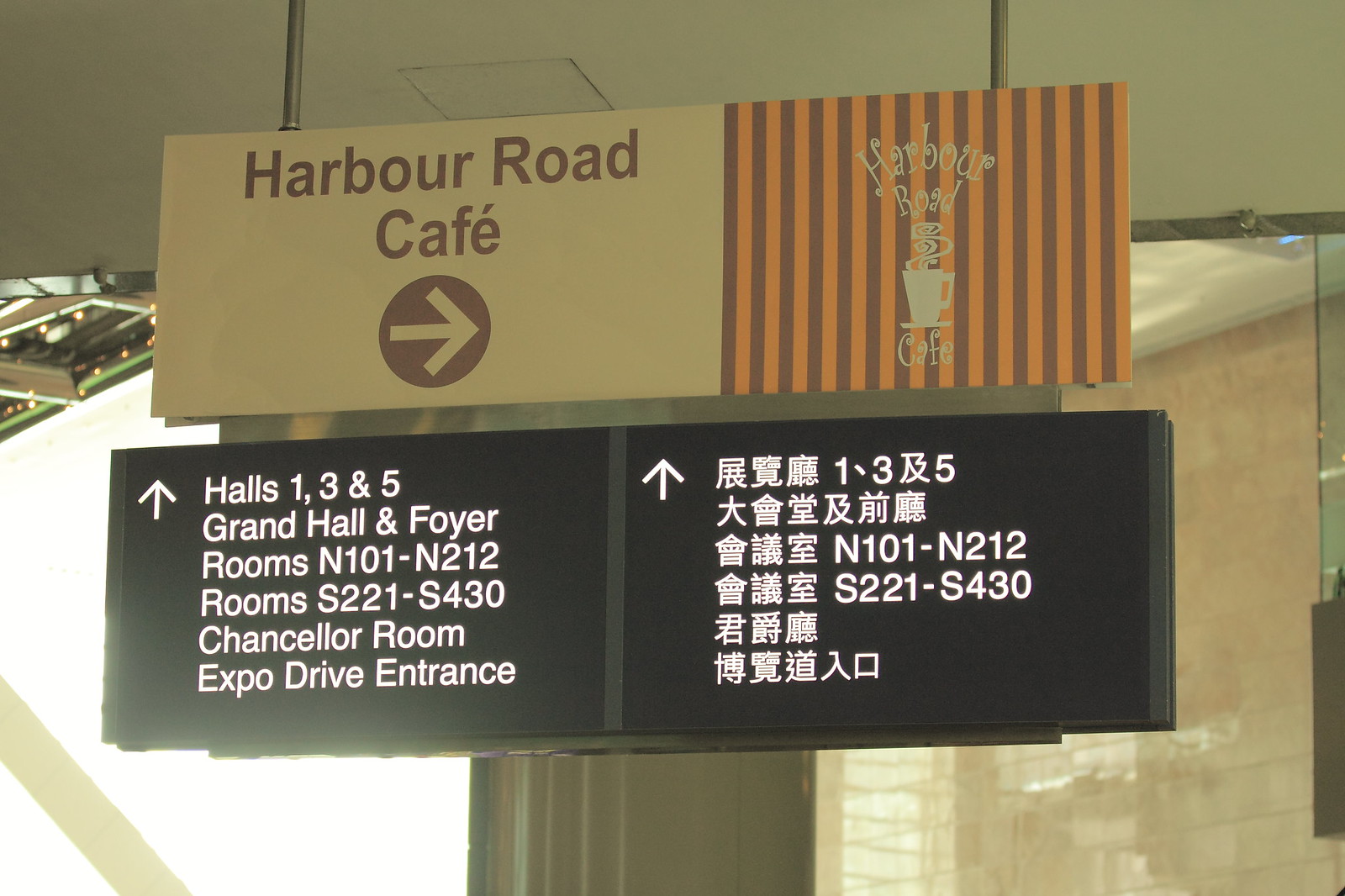The image depicts a full-color picture of signs hanging from a ceiling, likely in an indoor space, with windows visible in the background. The top sign features a cream-colored background with brownish text and a right-pointing arrow, indicating "Harbor Road Cafe." Adjacent to this is a section with orange and brown vertical stripes, also stating "Harbor Road Cafe" in white text and a steaming coffee cup logo. Below these signs is a black sign with two sections. The left side, in English with an upward-pointing arrow, lists "Halls 1, 3, and 5," "Grand Hall and Foyer," "Rooms N101-N212," "Chancellor Room," and "Expo Drive Entrance." The right side of the black sign provides the same directional information in Chinese, also with an upward-pointing arrow. The surrounding walls appear to be marble, and there are poles visible, suggesting a sophisticated, possibly hotel-like, environment.